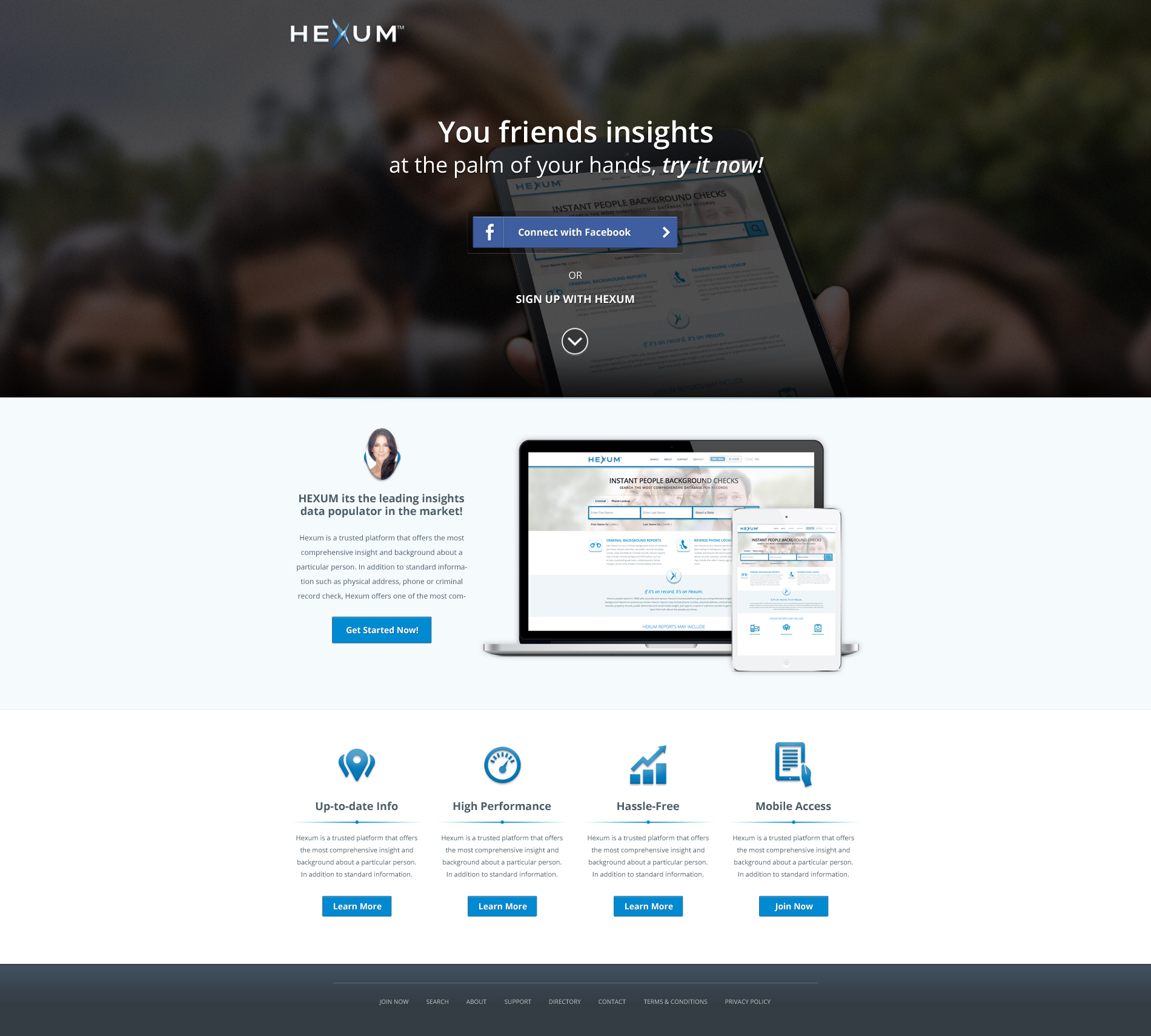Homepage of Hexum Website

The homepage of the Hexum website features a visually striking and modern design centered around their unique visual logo, which prominently displays two blue streaks forming the character 'X'. At the top of the page, visitors are greeted with a banner that offers options to connect with Facebook or sign up directly with Hexum, the latter being presented as plain text.

Additionally, a down arrow invites users to scroll down for more information. Below the banner, a clean layout presents details about Hexum’s offerings, accompanied by a stock image of an Apple laptop to reinforce the professional and tech-savvy vibe of the site.

Key information displayed includes a noticeably large text line stating, "Hexum is the leading insights data populator in the market." This is supported by a series of icons and descriptors emphasizing the platform’s core features such as up-to-date info, high performance, hassle-free operation, and mobile access. Each feature is associated with a clickable button for users to either learn more or join the platform, facilitating an engaging and user-friendly experience.